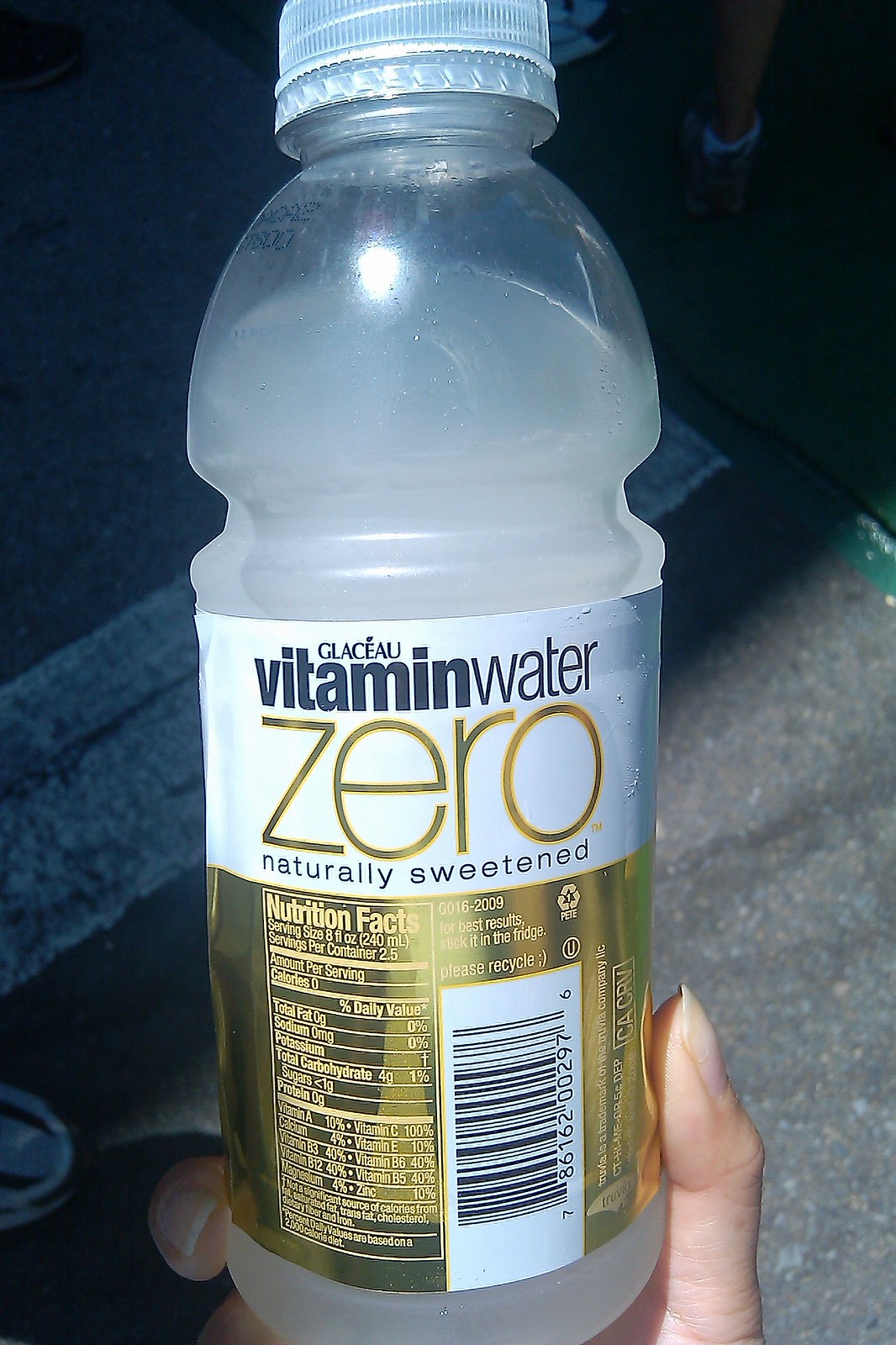This is a first-person POV photograph taken vertically, most likely on a phone, featuring a person holding a mostly full (approximately four-fifths) bottle of Vitamin Water Zero. The bottle is clear plastic with a white and gold label, prominently displaying the words "Vitamin Water Zero" in large gold font, along with "Naturally Sweetened" beneath it. It spans the entire vertical length of the image, centered and covering from top to bottom.

The bottle is being held in what appears to be the person's right hand, with their thumb and forefinger wrapped around its neck. The person seems to have long fingernails, suggesting they might be a woman. The photograph is taken outdoors on what looks like a road or pavement, indicated by visible white striping in the background.

Additional details include a clear white cap and black print around the neck of the bottle, potentially a best before date. The label is divided into white for the top third and a goldish chrome base for the bottom two thirds. The nutrition facts detail a serving size of 8oz or 240ml, totaling approximately 750ml for the entire bottle. Key nutritional information includes 0g total fat, 0mg sodium, 1% daily value of potassium, 4g total carbohydrate (1% daily value), less than 1g sugar, and 0g protein. The label also lists several vitamins: A, C, E, B6, B5, and zinc, along with other vitamins that are not clearly readable. Other notable aspects include the barcode situated on the right side of the nutrition facts.